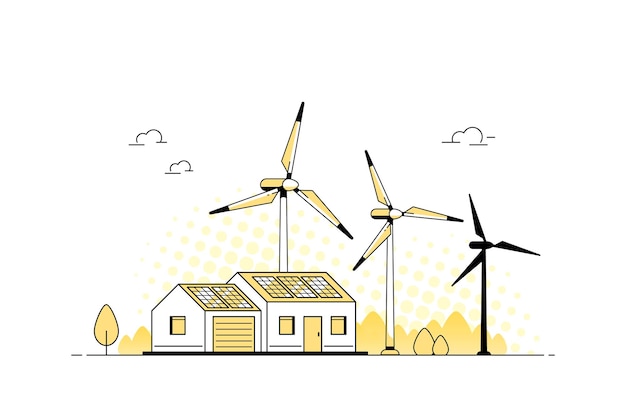This minimalistic, stylized cartoon illustration depicts a simple home with an attached garage, highlighted against a white background dotted with clouds. The house is equipped with five solar panels on its roof, emphasizing its reliance on renewable energy. Next to the home, three modern wind turbines with triangular blades contribute to the generation of electricity, possibly for the home or the surrounding neighborhood. Additional details include a lone tree to the left of the house and some bushes beside it. The entire scene is rendered in a palette of yellow, black, and white, with yellow splashes and dotted gradients adding subtle depth to the background.